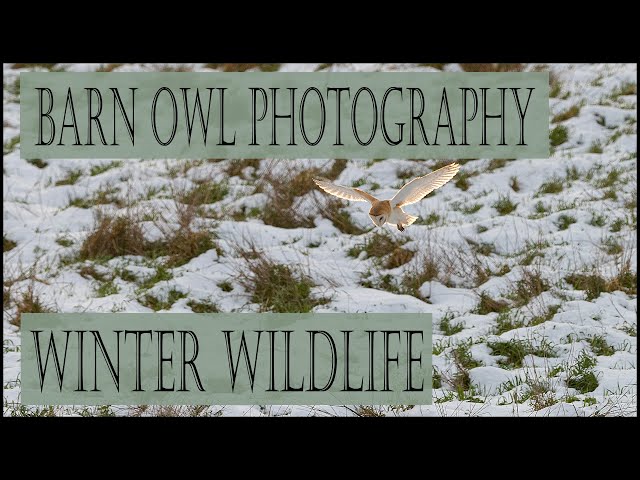This advertisement features a striking photograph of a snowy, grassy field with tufts of green and brown vegetation emerging through the snow, suggesting either fresh snowfall or melting snow. Dominating the center of the image is a majestic barn owl in mid-flight. The owl's body is predominantly white, with light brown markings on its head and the base of its wings, and dark black feet. Its wings are outstretched, and it appears to be scanning the ground, possibly in search of prey. The image is set in a landscape orientation, framed by thick black stripes at the top and bottom. Two light green bars with black text are superimposed on the photograph; the top bar reads "Barn Owl Photography" and the bottom bar reads "Winter Wildlife," covering approximately 30% of the image. The entire scene is backlit, highlighting the owl’s features and adding depth to the snowy landscape.